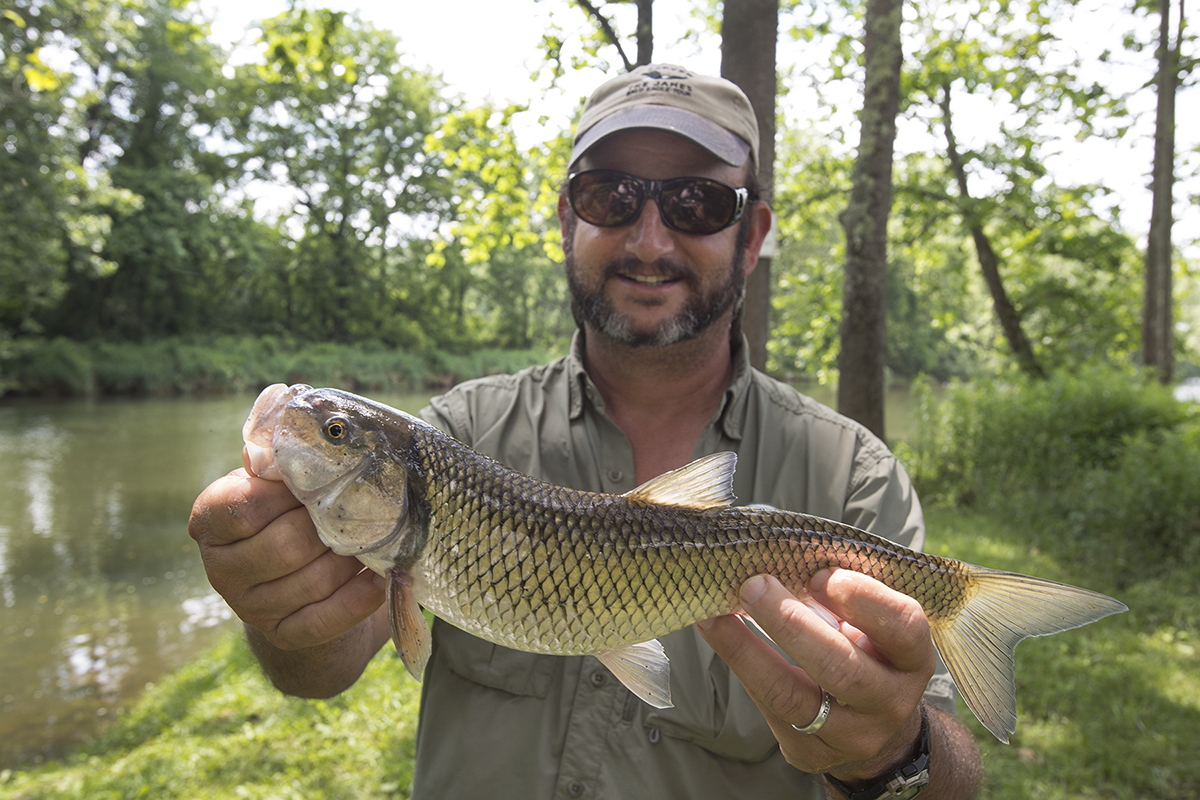The image captures a proud fisherman standing at the center, holding out a sizable bass with both hands—the head in his left and the tail in his right. The man has brown skin, a black and gray peppered beard, a mustache, and sideburns. He is clad in a short-sleeved, dark gray button-down shirt, black sunglasses, and a light gray baseball cap. A silver ring adorns his left finger, accompanied by a black watch on his left wrist. The fish he holds boasts a myriad of colors: a dark gray top, transitioning to a light green body, and ending with a dark green tail. Its mouth, supported by the fisherman’s hand, has white and pink hues, with yellow eyes and black pupils. Surrounding this central figure is a picturesque, wide vertical scene featuring a curving, murky green river bordered by green grass and lush trees with brown trunks and green leaves. The background reveals a vibrant blue sky with scattered white clouds, bathing the scene in warm sunlight.